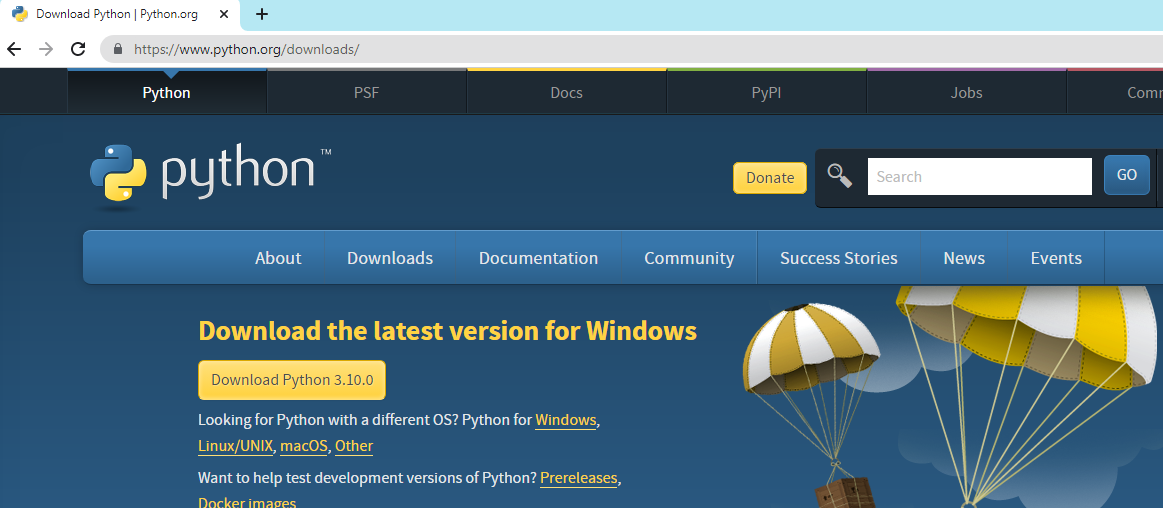A screenshot captured from the Python.org website, specifically the Download section at python.org/downloads. The website's top banner features a dark gray background, complemented by a submenu that includes options such as Python, PSF, Docs, PyPI, Jobs, and more. The main content area of the page is predominantly blue. Positioned at the top left, adjacent to the word "Python," is the site's logo, which resembles a yellow and blue stylized plus sign.

Beneath the primary navigation, there is a submenu highlighted in a lighter blue shade, offering various clickable options: About, Downloads, Documentation, Community, Success Stories, News, and Events. Prominently displayed is a call-to-action to "Download the latest version for Windows," followed by a section that reads, "Download Python 3.10.0." This section lists the available platforms: Windows, Linux/UNIX, MacOS, etc., and mentions Docker images associated with the pre-release versions.

Every element is meticulously organized, providing users with precise information and easy access to the tools they need.